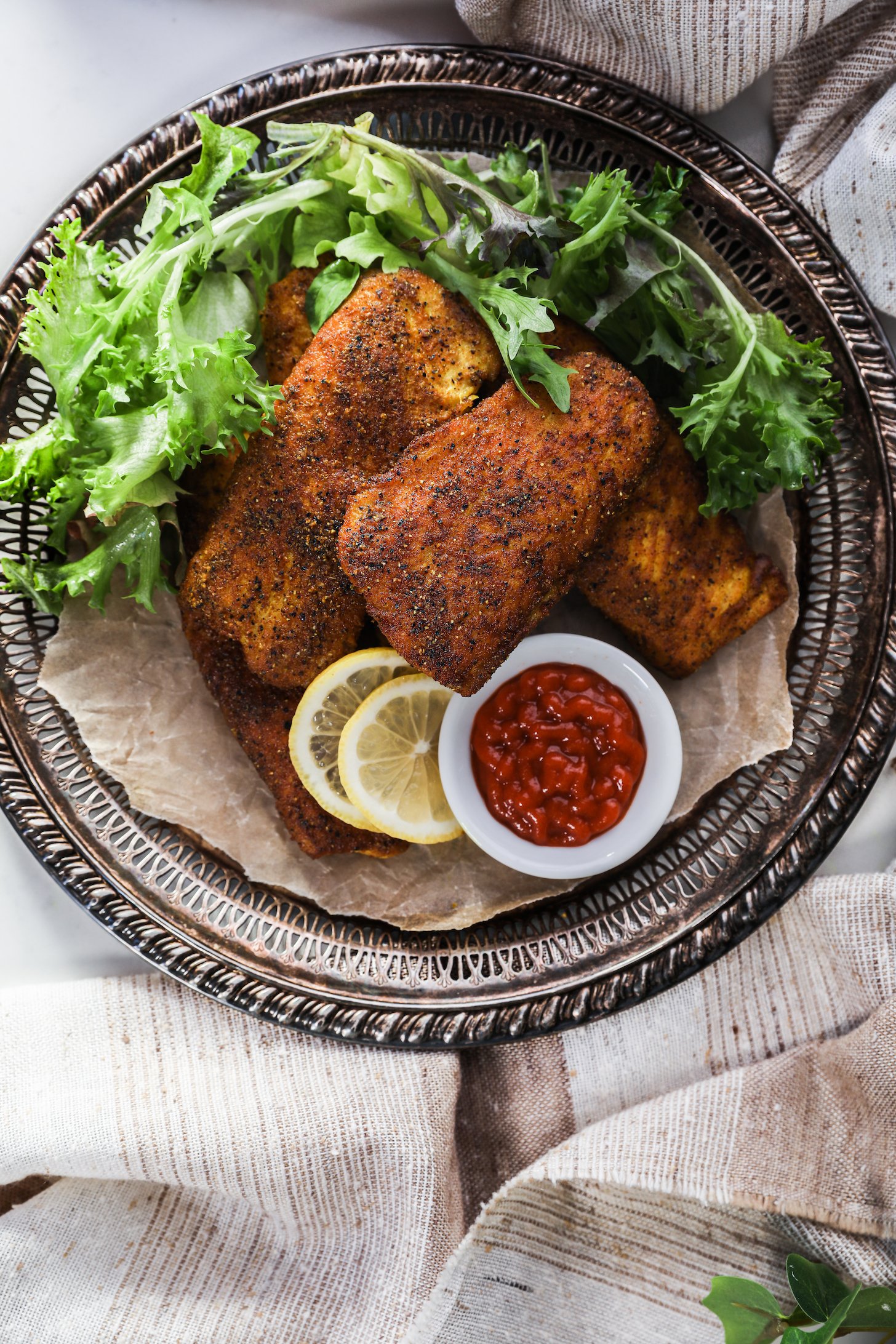This image showcases a meticulously arranged dish set on a round, metallic plate with a brass hue and a braided design along the outer edge, resting atop a combination of white and tan striped linen napkins. The centerpiece is four well-cooked pieces of chicken, possibly fried, exuding a rich brown and orangey coating that suggests a flavorful preparation. Two lemon slices adorn one of the chicken pieces, adding a vibrant contrast. Surrounding the chicken, fresh, green romaine lettuce enhances the visual appeal and hints at added freshness. In the foreground, a small, white dipping bowl features a vibrant red sauce, likely ketchup. Additionally, a piece of wax paper is placed underneath the chicken, and a small sprig of leafy greens occupies the bottom right corner of the composition, completing this appetizing presentation.